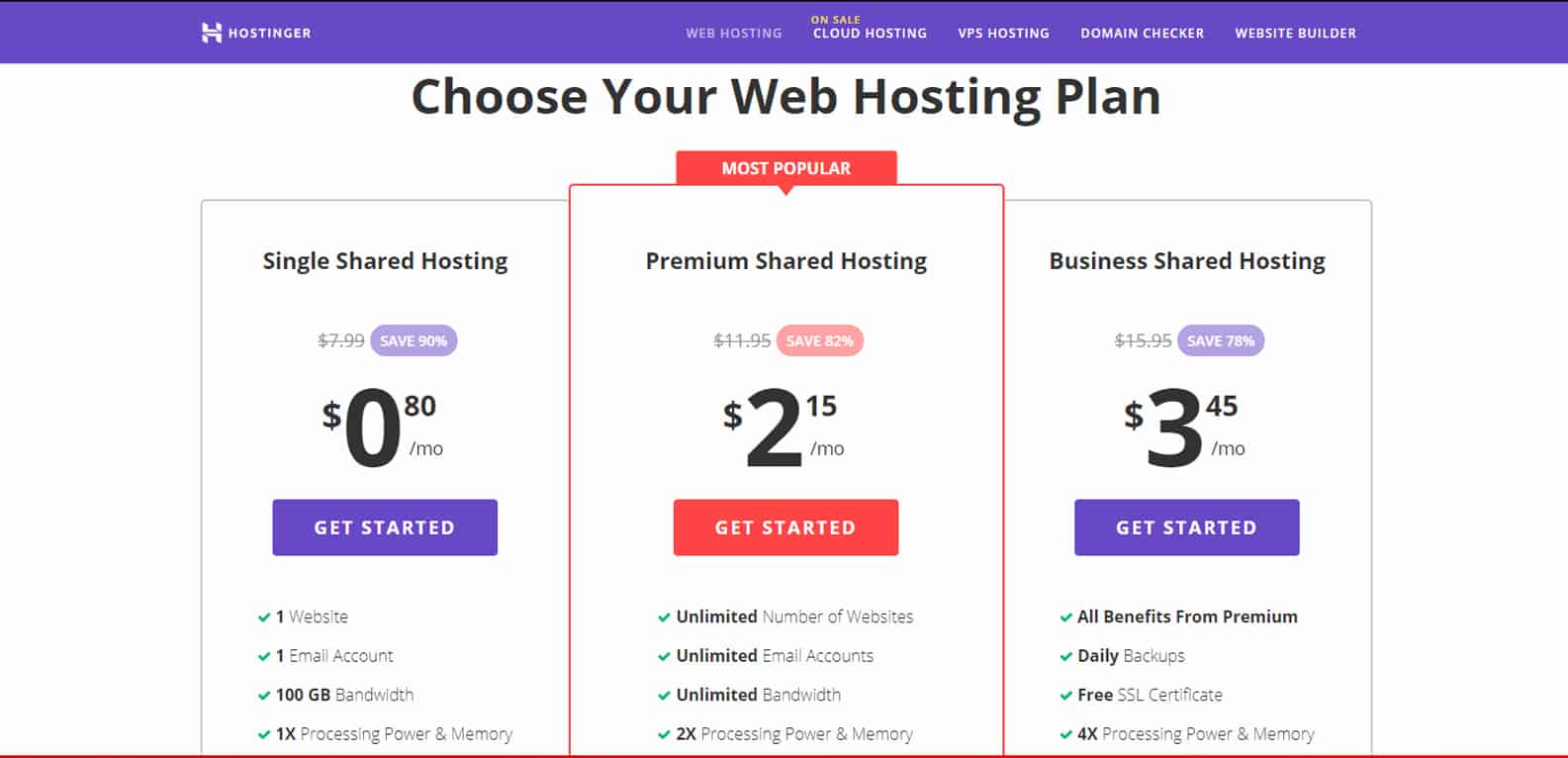The image depicts a detailed screenshot of web hosting plans from a hosting website. The top portion of the screenshot features a purple banner. Below, the main section, set against a white background, displays three distinct pricing plans in separate boxes. 

**Left Box:** 
- **Color:** Purple 
- **Plan:** Single Shared Hosting
- **Price:** $0.80 per month
- **Features:** Website, Email, 100 GB of bandwidth
- **Call to Action:** "Get Started"

**Center Box:** 
- **Color:** Red (highlighted as "Most Popular")
- **Plan:** Unlimited Hosting 
- **Price:** $2.15 per month
- **Features:** Unlimited resources across the board
- **Call to Action:** "Get Started"

**Right Box:**
- **Color:** Purple
- **Plan:** Business Shared Hosting
- **Price:** $3.45 per month with a note that this price reflects a 70% savings when paid annually
- **Features:** All benefits, daily backups, free SSL certificate
- **Call to Action:** "Get Started"

At the bottom, there is a white space with the text "Choose your web hosting plan," indicating the option to choose and compare plans, with an emphasis on annual payment plans.